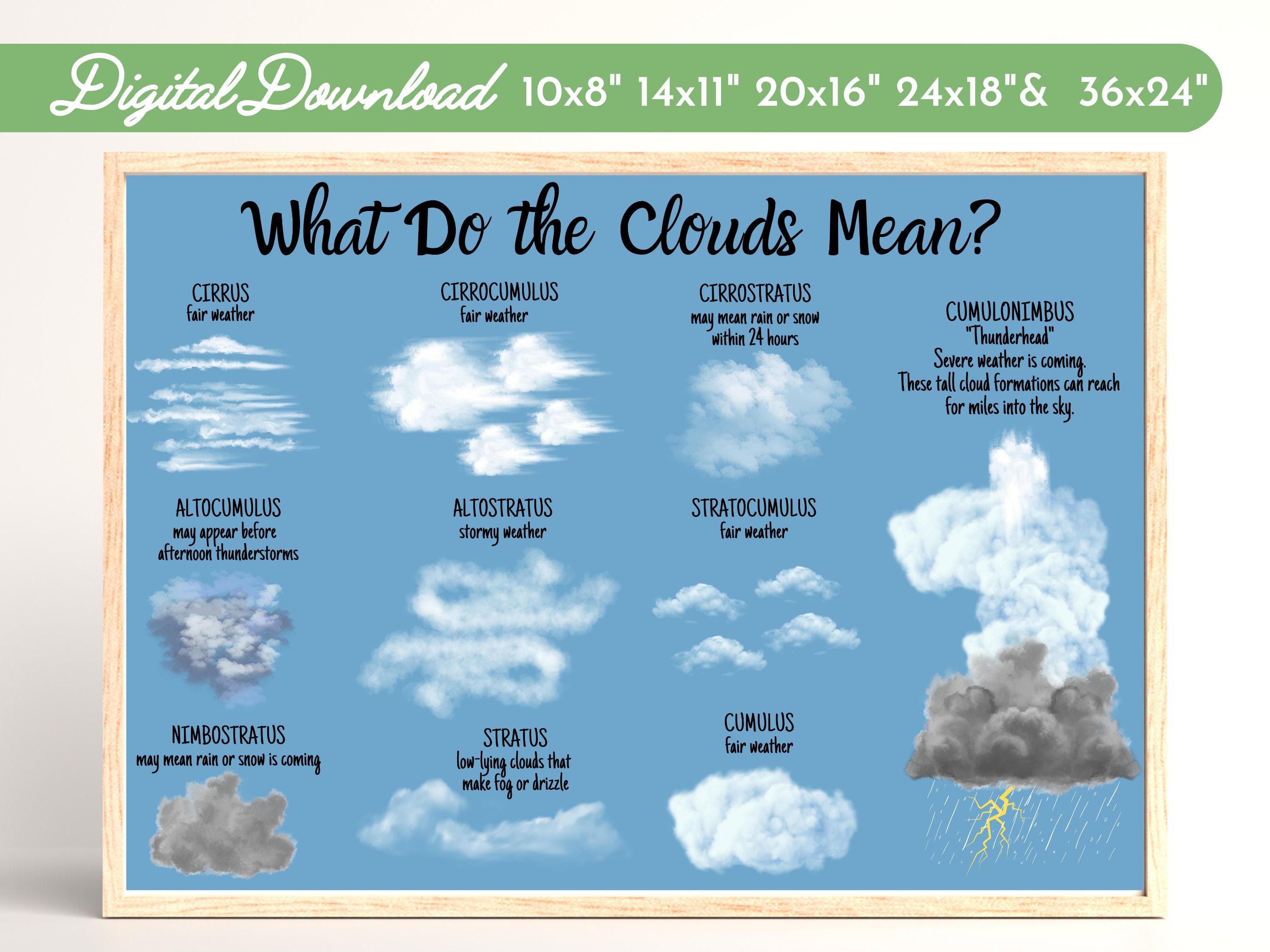This image displays a detailed, computer-generated poster titled "What Do The Clouds Mean?" framed in light oak wood. The background is a serene sky blue, and the title is elegantly written in cursive black font. Above the poster, a green banner with rounded ends announces, "Digital Download," available in various sizes: 10x8 inches, 14x11 inches, 20x16 inches, 24x18 inches, and 36x24 inches.

The poster features twelve types of clouds, each depicted with corresponding illustrations and descriptions of the weather they signify. The clouds are organized in rows, starting with:

1. **Cirrus** - Fair weather, illustrated as thin, wispy clouds.
2. **Cirrocumulus** - Fair weather, shown as larger, poofy clouds with wisps.
3. **Cirrostratus** - May indicate rain or snow within 24 hours, depicted with a blue-green tint.
4. **Altocumulus** - May appear before afternoon thunderstorms, illustrated as white clouds with hints of purple.
5. **Altostratus** - Indicative of stormy weather, depicted as thin, circular clouds with blue centers.
6. **Stratocumulus** - Fair weather, shown as four puffy white clouds.
7. **Nimbostratus** - May mean rain or snow is coming, depicted as a large, brown cloud.
8. **Stratus** - Low lying clouds that create fog or drizzle, illustrated in greenish-blue.
9. **Cumulus** - Fair weather, shown as white puffy clouds resembling cotton balls.

In the final column on the right is the **Cumulonimbus** or "Thunderhead," which signifies severe weather. This cloud is illustrated transitioning from a white, puffy top to a dark gray base with rain and lightning bolts emerging, indicating its towering, storm-bringing nature.

This poster serves as an educational tool, blending aesthetic appeal with practical meteorological information.